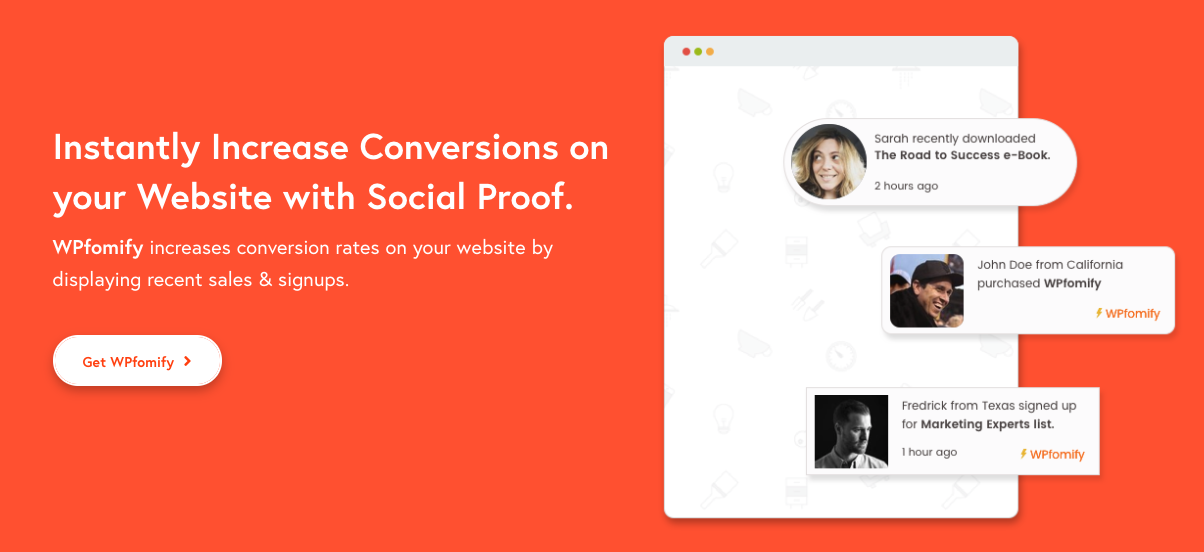This image appears to be a professionally designed advertisement for the WPFOMIFY plugin, displayed on a website. The advertisement features a solid orangish-red background that creates a striking contrast with the prominently displayed white text on the left side of the image. The caption reads, "Instantly increase conversions on your website with social proof." Below that, in smaller text, it says, "WPFOMIFY increases conversion rates on your website by displaying recent sales and sign-ups."

To the right of the text, there's a call-to-action button labeled "Get WPFOMIFY," inviting viewers to engage with the product. Beside the button, three profile images illustrate the concept of social proof:

1. A circular image of a blonde woman named Sarah, with an accompanying text stating, "Sarah recently downloaded the Road to Success e-book two hours ago."
2. A profile picture of a white man wearing a baseball cap, identified as John Doe from California, with a caption indicating he "purchased WPFOMIFY."
3. A black-and-white profile photo of another white man named Frederick from Texas, with text noting that he "signed up for a marketing experts list one hour ago." 

The carefully curated profile images and timestamps aim to demonstrate how WPFOMIFY can enhance website credibility and boost conversion rates by leveraging recent user activity to attract new customers.